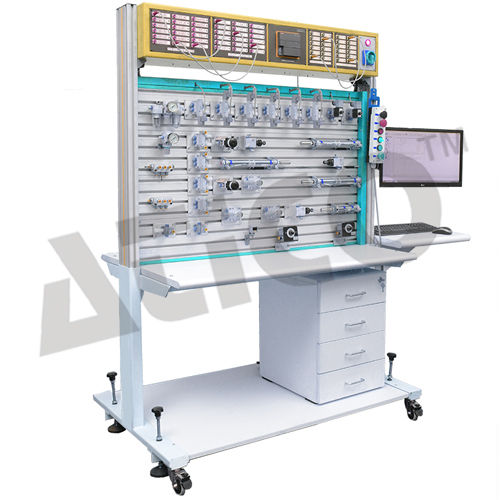The image depicts a mobile, hospital-like medical cart with a white base, supported by four black wheels and stabilizers for stationary use. The cart features a bottom shelf with white layers and a brown-teal bordered structure for added support and stability. Attached to the right side of the cart are four removable white drawers, ideal for storing various items.

Above the drawers, the cart houses an intricate electronic system, featuring a prominent circuit board-like component in yellow and brown hues, festooned with numerous buttons, knobs, and interconnecting wires. This electronic setup appears to be connected to a white platform, suggesting it might serve a specialized function.

On the right side of the cart, a pull-out shelf supports a computer setup, including a monitor, keyboard, and mouse, likely providing a user interface for the electronic system. The entire apparatus is framed against a white backdrop, and the photograph bears a watermark featuring a triangle with the letters "C-I-C-O" or "A-T-I-C-O" in gray text.